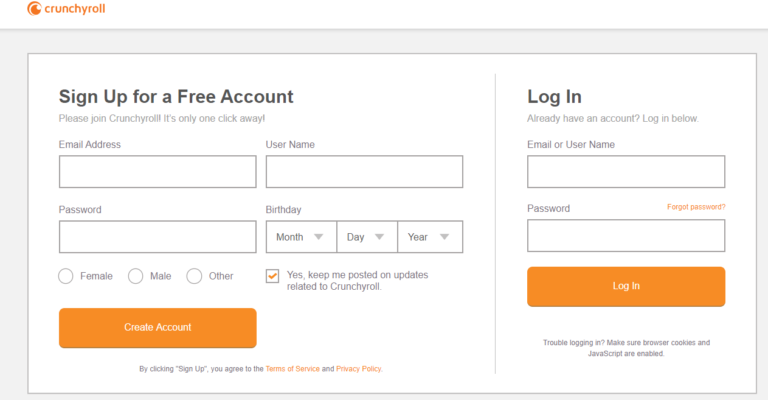Screenshot of the Crunchyroll Account Signup Page

The image displays a screenshot of the Crunchyroll account signup page. At the top left corner, you see the Crunchyroll logo in a combination of orange, black, and white colors. Below the logo, there is a prominent white box with the title “Sign Up for a Free Account” in bold text.

The signup form requires the following details:
- Email Address
- Username
- Password
- Birthday (with separate fields for month, day, and year)
- Gender selection (options include Female, Male, or Other)

Additionally, there is a checkbox with an orange checkmark labeled “Yes, keep me posted on updates related to Crunchyroll.” At the bottom of the form is an orange “Create Account” button with white text. Below the button, a note specifies that by clicking “Sign Up,” you agree to the Terms of Service and Privacy Policy, with both the Terms of Service and Privacy Policy text in orange, making them easily identifiable and clickable.

For users who already have an account, there is an alternative login section. This part includes fields for entering your email or username and password. Next to the password field, there’s an orange “Forgot Password?” link, providing an easy way for users to reset their password if necessary. The “Login” button is also in orange with white text. 

A footer note advises users facing login issues to ensure that their browser cookies and JavaScript are enabled, though the use of JavaScript for login credentials is humorously critiqued as an outdated practice. 

Overall, the screenshot captures both the signup and login functionalities of the Crunchyroll web page in a straightforward and user-friendly layout.